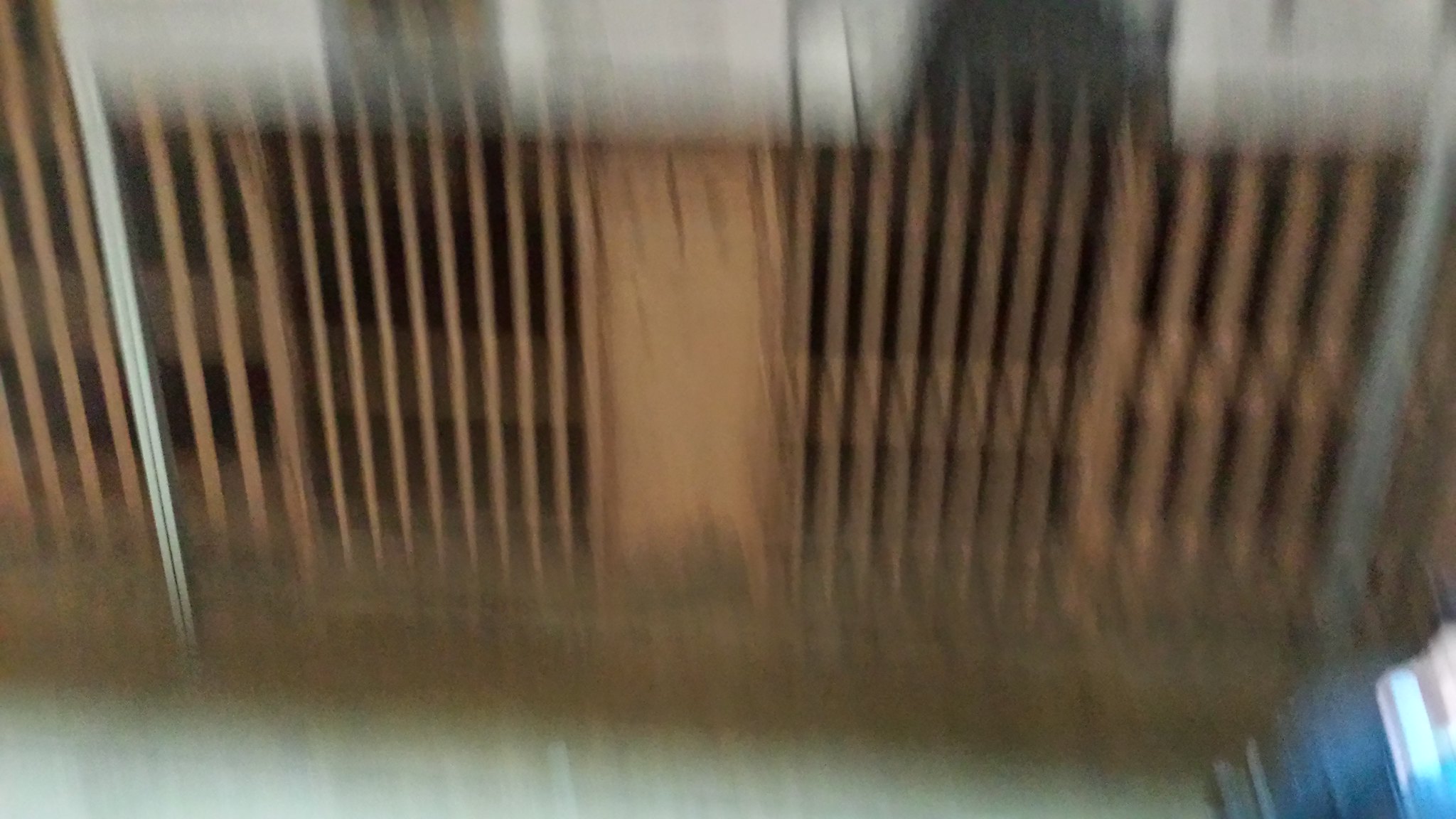This image is extremely blurry, making it difficult to determine exactly what it depicts. The predominant elements are a series of vertical brown lines covering the midsection, which resemble a brownish or bronze-colored gate with numerous spikes running horizontally across the frame. Surrounding these lines are various shades of brown, suggesting either a fence or stacked boards. The top section features blocks of gray with a black corridor-like segment in the upper middle. There are two gray metal pieces, one in the upper right and one extending to the bottom, potentially indicating a hinge or joint. At the lower right, there's a dark blue area with a white streak, next to a section of gray floor. At the very bottom left, there's additional white coloring across the image.